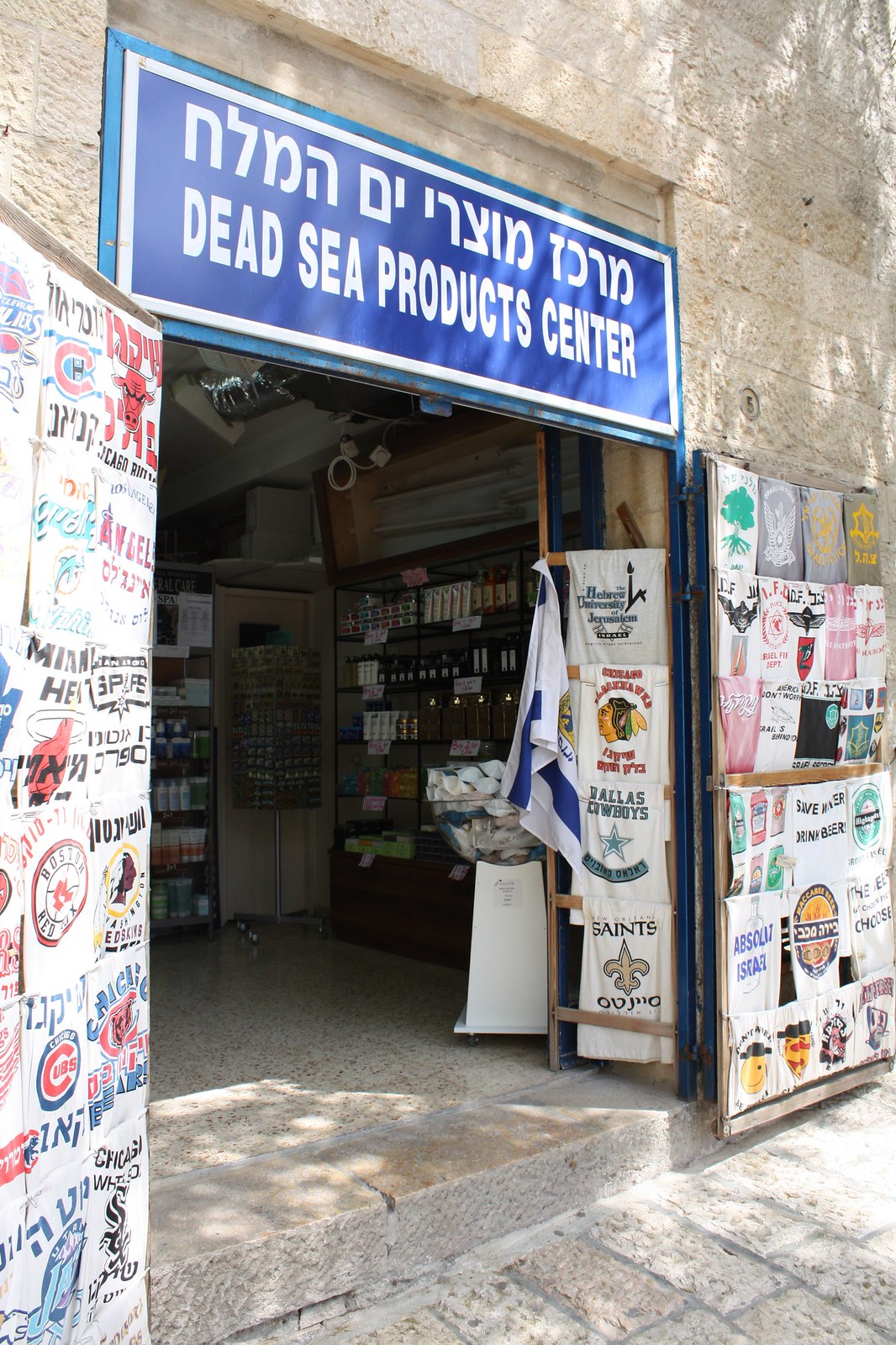The image features the exterior of a brick-built store, with sand-colored bricks and an arching open entrance that allows a glimpse into the dimmer interior. Situated above the entrance is a blue sign with white framing, displaying text in a Middle Eastern script alongside the English words, "Dead Sea Product Center." The shop specializes in selling various items, prominently displaying t-shirts and sports jerseys. Hanging from the left side of the entrance are t-shirts featuring the Chicago Bulls, while the right side showcases jerseys for the New Orleans Saints and the Dallas Cowboys. Inside, more t-shirts are visible, adding to the impression that the store has a focus on apparel. The brighter daylight outside contrasts with the darker interior, hinting at a variety of other products within, possibly including drinks visible in the background.